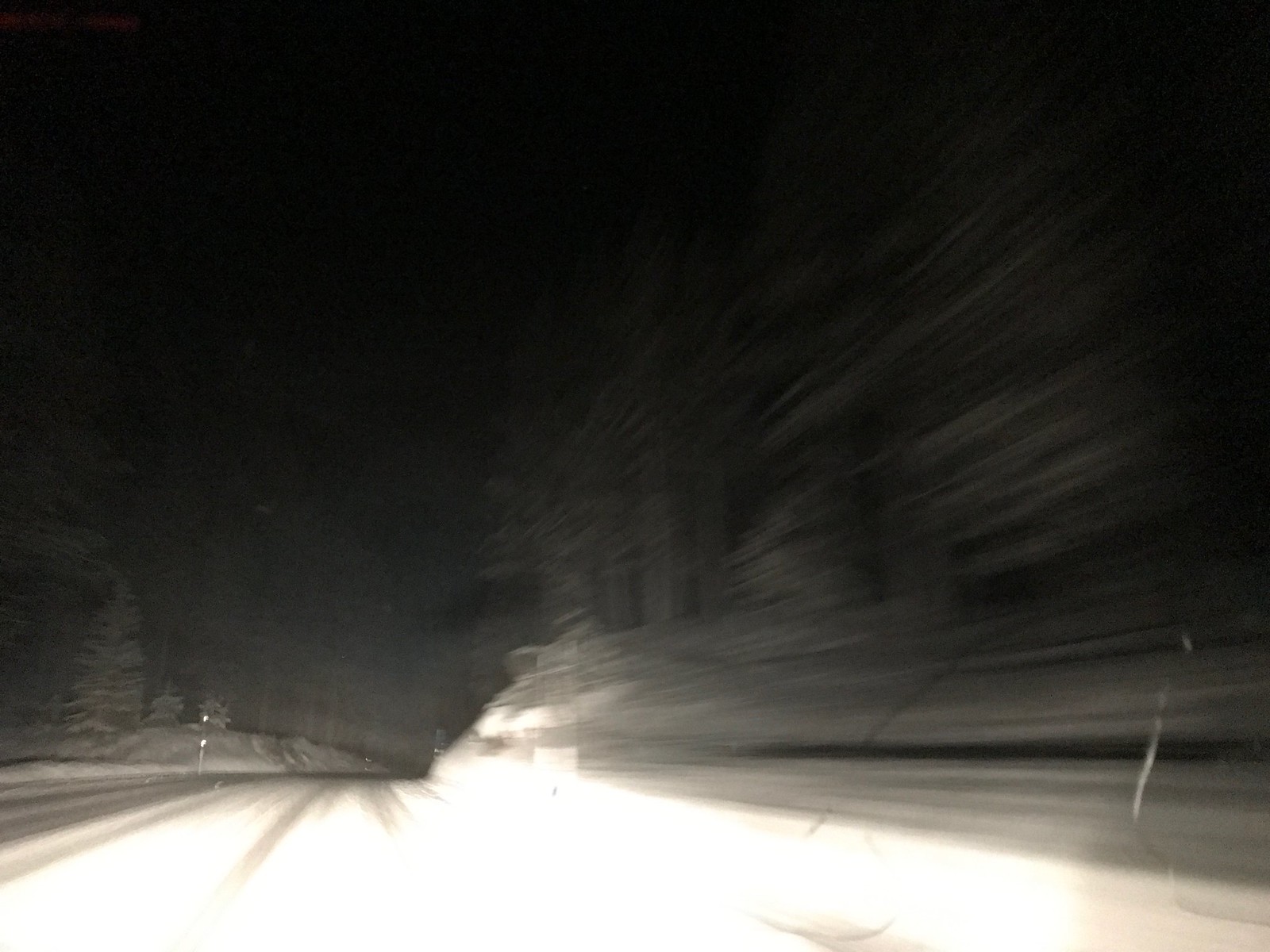This evening photograph, likely taken through a car window, captures a vehicle in motion on a snow-dusted road, amplified by the blurred effects characteristic of long-exposure photography. The scene is enshrouded in darkness, with an expansive black sky dominating the frame. The vehicle’s headlights illuminate the road ahead, casting a bright light that reveals a snowy landscape along the roadside, particularly noticeable on the left side where a hill appears covered in snow. The right side of the image suggests the presence of trees or buildings, though they are less distinct due to the blurred effect, further emphasizing the vehicle's speed and motion. The overall impression is one of dynamic movement, a nighttime journey through a wintry, tree-lined path.